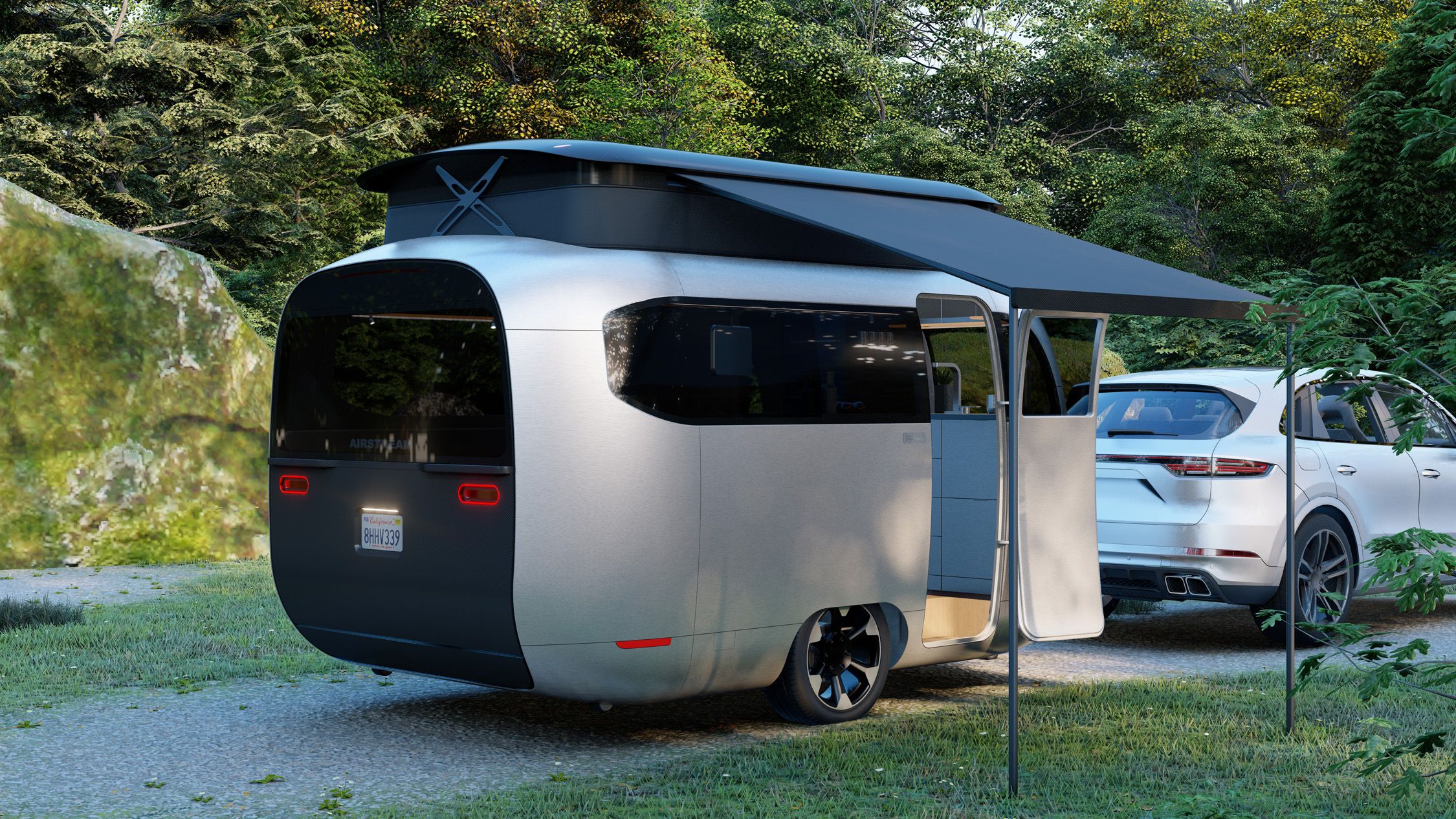The photograph captures a sleek, silver, and rounded camper trailer with a futuristic design, attached to a white four-door SUV. The camper trailer features a large extended roof that pops up and a black canopy awning attached to a sturdy metal frame. The awning extends from the roof and is supported by two poles resting on the ground. The camper's side door is open, partially revealing the interior, and it has tinted windows running along its sides, front, and back. At the rear of the camper, two red, oval-shaped brake lights are visible, along with a white license plate marked "AHHV339" in blue text. The camper, which has one visible black rubber wheel with a white rim, is parked on a gray gravel-like road, bordered by green grass. The background includes a natural setting with trees, a moss-covered rock, and a serene, wooded area.